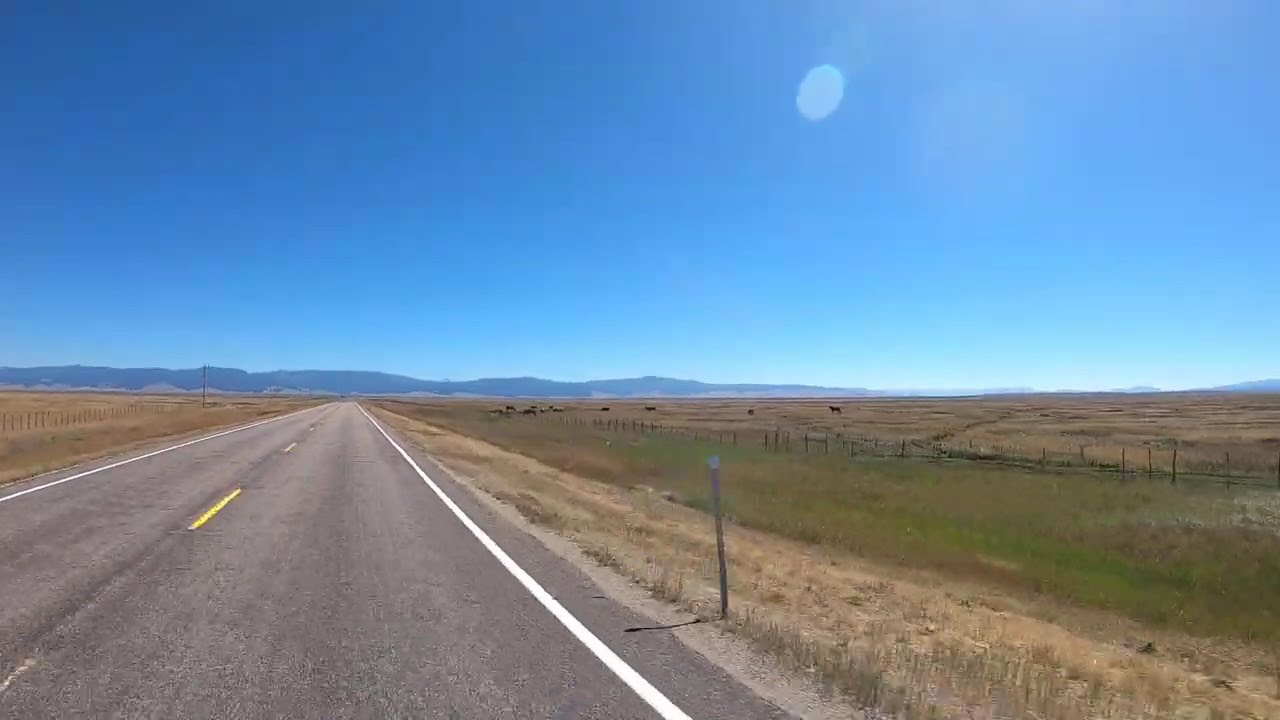The image depicts a scene set on a two-lane paved road during a bright, sunny day. The road, positioned towards the right-hand side of the frame, features white solid lines on the outer edges and a yellow dotted line down the center, emphasizing its narrowing perspective. To the right of the road lies an expansive field enclosed by a fence, where a herd of animals, possibly cows, graze in the distance. On the left side, another fenced-off field displays a predominantly light tan color, suggesting a wheat field, with a narrow strip of green. A milepost marker is visible nearby. The top half of the picture is dominated by a vivid blue sky, marred only by a round, lighter blue spot that might be a lens distortion or a smudge. Along the midline horizon, far-off hills or mountains rise, contrasting with the mainly brownish ground cover that hints at a late season or an area not fully greened up.